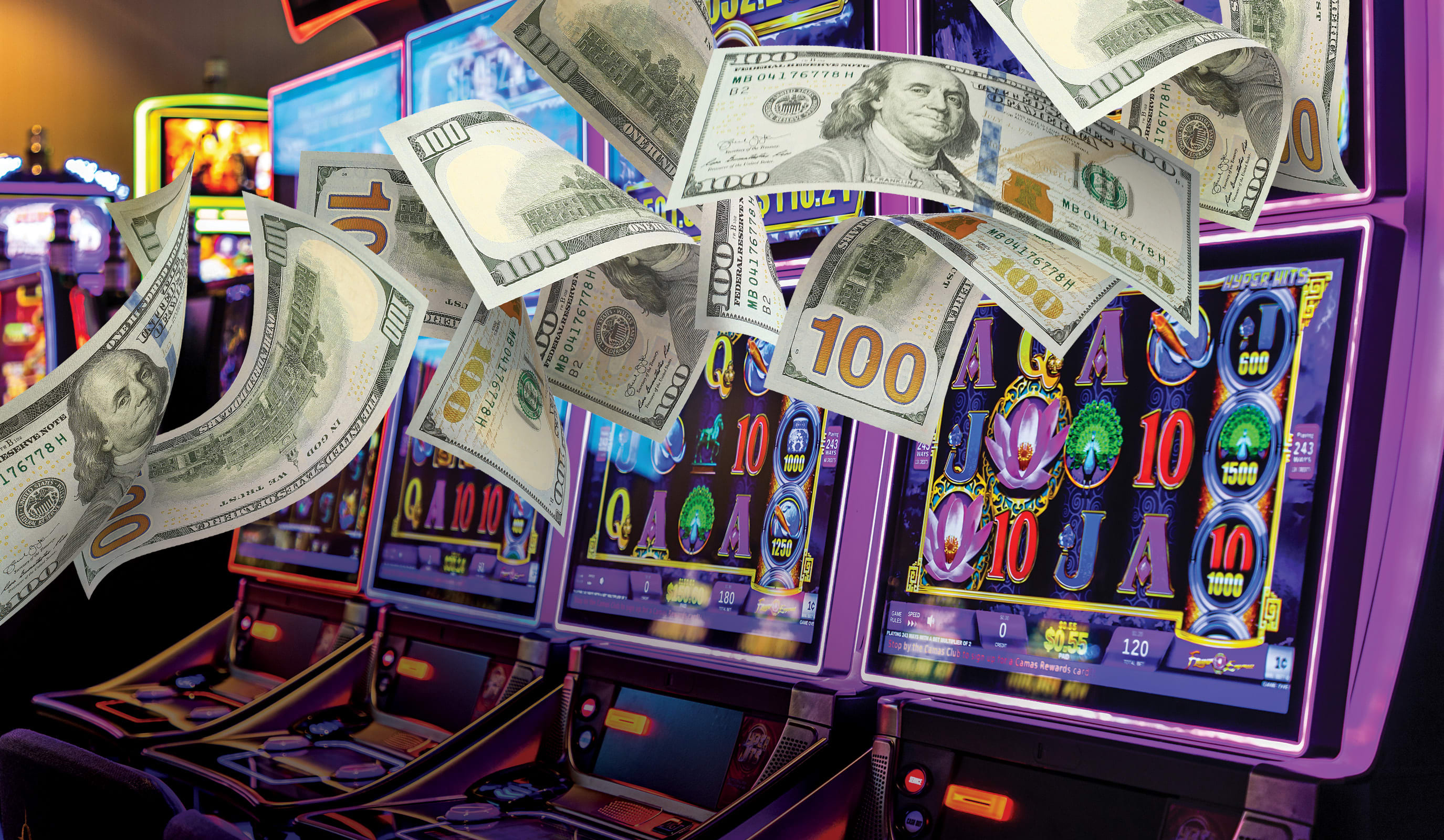This detailed image captures the vibrant and electrifying atmosphere of a casino. In the foreground, four vividly illuminated, purple slot machines are prominently displayed. Each screen is a colorful array of symbols including 10s, Jacks, Queens, and Aces in hues of red, blue, and yellow, alongside other icons like lotus flowers and peacocks. Overlaid digitally across the scene are multiple $100 bills, featuring Benjamin Franklin's likeness, seemingly airborne, adding a sense of dynamic motion as they scatter from left to right. These notes appear to be flying closer to the camera, creating a layered, depth-filled effect. In the background, additional blurred machines can be seen, suggesting a dense, indoor setting filled with a multitude of gaming options. The slot machines are distinctly marked by buttons in place of traditional pull triggers, further emphasizing their modern, digital nature.